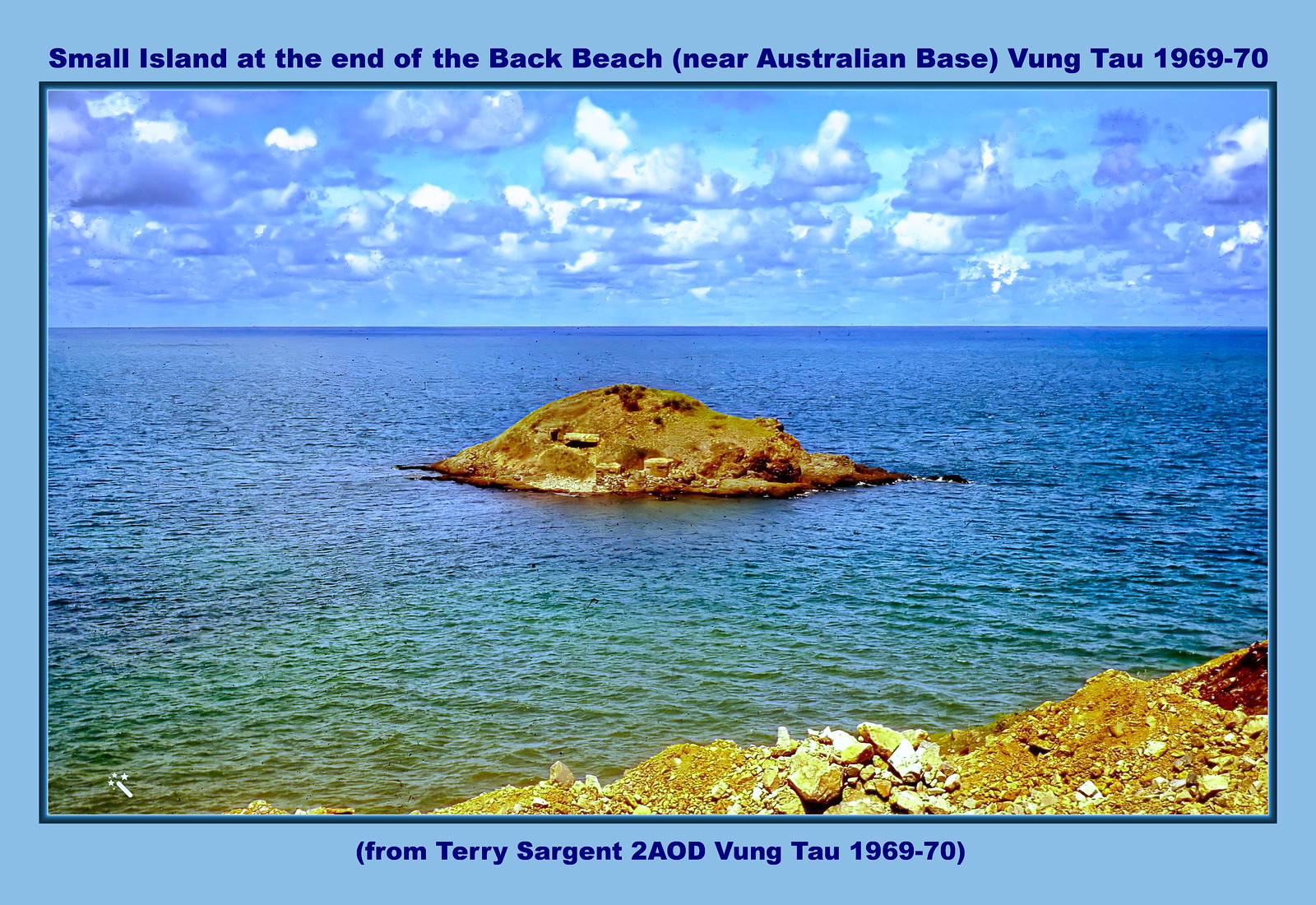The image resembles a vintage postcard, featuring an ocean view with a small landmass or large rock near the horizon, resembling an island. The scene is framed by a thin black border and a thicker solid blue border. At the top of the photo, blue text reads "Small island at the end of Back Beach near Australian base Vung Tau 1969-70," while the bottom includes a parenthetical note: "From Terry Sergeant, 20 AOD Vung Tau 1969-70." The ocean stretches from a rocky, seaweed-dotted shore in the lower right, where the water transitions from a greenish hue near the shore to a deeper blue further out. Above, the sky is filled with puffy white clouds against a blue backdrop, capturing the serene beauty of the seascape.